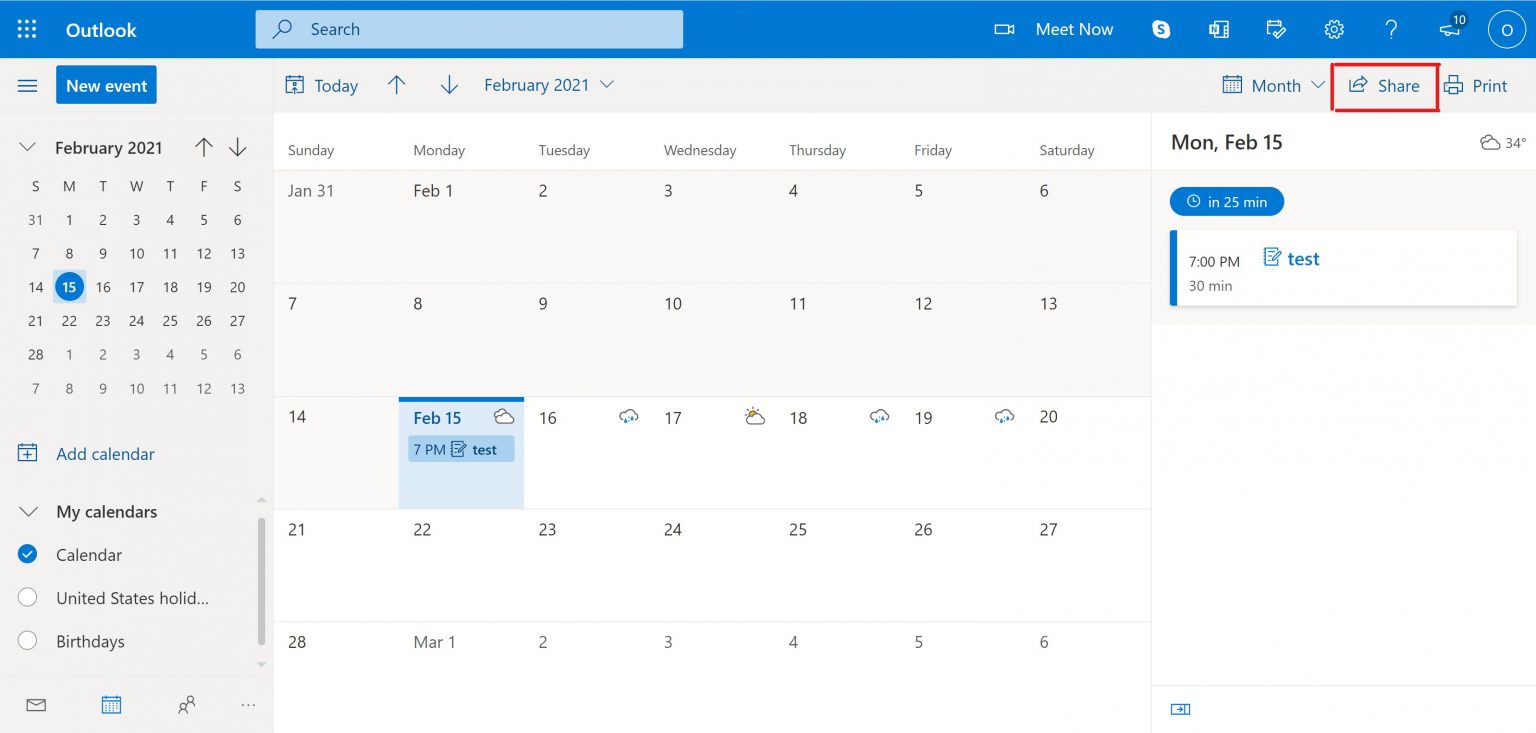The image depicts a detailed view of a digital calendar for February 2021, displayed in a Microsoft Outlook interface. At the top of the image, there is a long blue bar with the word "Outlook" on the left and a search bar featuring a magnifying glass icon on the right. Below this, there's another bar with a prominent blue square labeled "New Event" on the left. On the right side of this bar, you'll find a set of controls including "Today," an upward-pointing arrow, a downward-pointing arrow, and the date "February 2021." 

Further to the right, there is a mini-calendar preview next to the word "Month," followed by the word "Share" inside a red-outlined square, and a "Print" option. 

In the main calendar view, the month and year "February 2021" are displayed on the left, with the date Monday, February 15th circled in blue. This date is highlighted again on the main calendar grid, marked with a blue color and the notation of an event at 7 p.m. called "test," indicated by a cloud icon.

At the bottom left, there is an option to "Add Calendar." Below this, under "My calendars," is a list including "Calendar" which is marked with a blue checkmark, "United States holidays" with a white circle next to it, and "Birthdays" also with a white circle beside it.